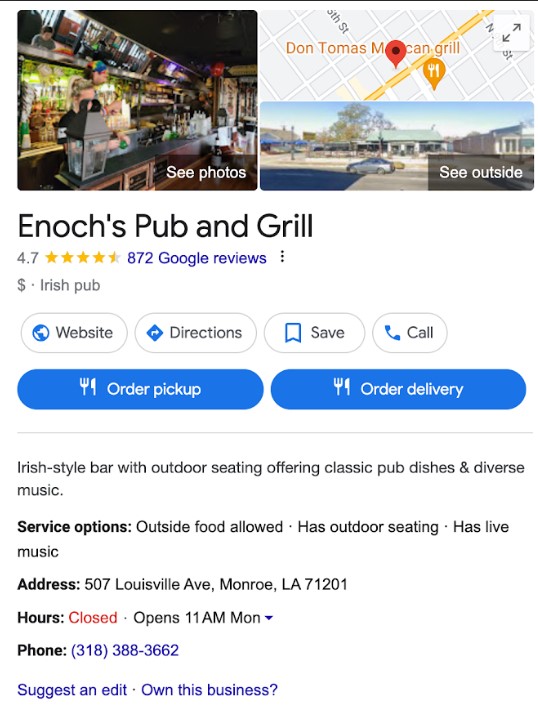The image depicts a partial screenshot of the front page of a Google search result, prominently featuring "Enoch's Pub and Grill." 

In the upper-left corner, an image showcases a bar scene with several mirrors or TVs mounted above the bar area. A small text overlay in the corner of this image reads "See photos." 

Adjacent to this image, the text reads "Don Thomas McKinn Grill, M." Nearby, an icon resembling a GPS marker appears, followed by the text "CAN Grill" which may refer to a potential Mexican Grill. 

Below this section, there is a small map indicating the location and a photograph that seems to capture the exterior of the establishment. A prompt in the bottom right corner of this photo says "See outside."

Underneath the images and map, the listing "Enoch's Pub and Grill" is displayed prominently, accompanied by a rating of 4.7 stars based on 872 Google reviews. Beneath this, buttons for "Website," "Directions," "Save," and "Call" are visible, along with additional buttons labeled "Order pickup" and "Order delivery," each marked by a fork and knife icon.

Further down, detailed information about the pub is provided, including its address, hours of operation, and phone number.